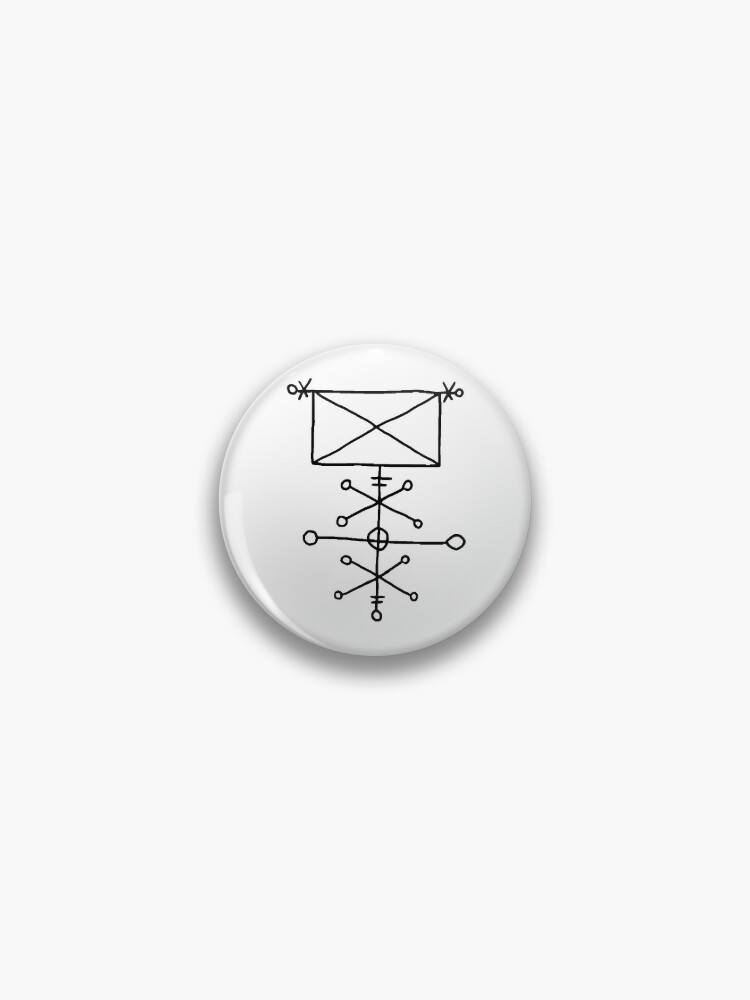The image features a round, white button with a black, esoteric diagram on it, resembling an intricate yet ambiguous schematic. The button is set against a featureless white background. The diagram on the button starts at the top with a rectangle crossed by an X. Emerging from this rectangle are various elements: two smaller Xs on either side, flanked by circles. Below, a long vertical line connects several components, beginning with two short parallel lines of varying lengths. Next, there's a large X with circles at its ends, followed by another line with circles at both ends and a circle crossing over its middle. Further down, there's another large X with circles at its points, and finally, at the bottom, the design concludes with two short lines and a single circle. The enigmatic design, possibly Kabbalistic or schematic-like, lacks any text, adding to its mysterious nature.